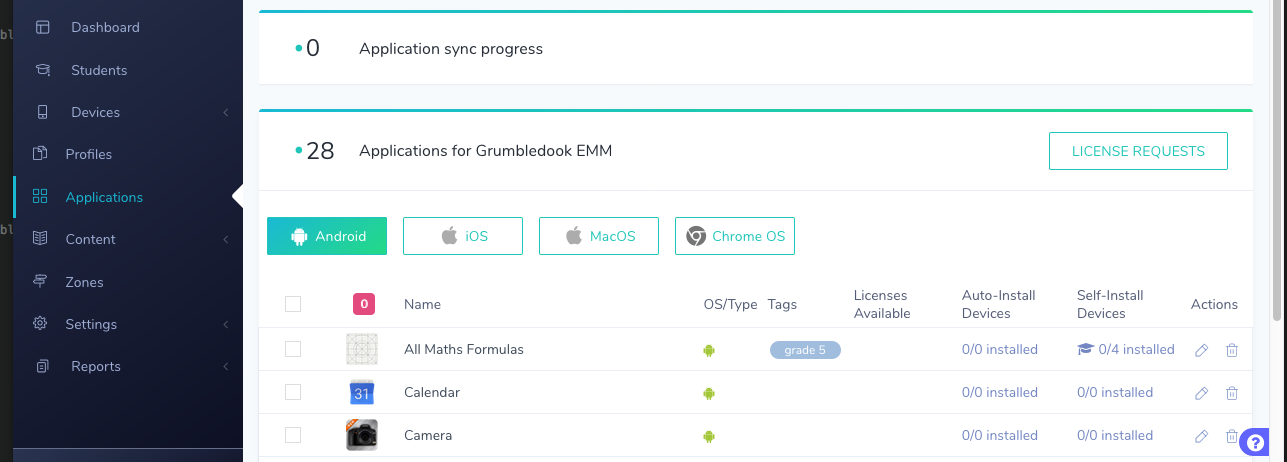The image is a horizontally rectangular partial screenshot from a software application. On the left side, there is a vertically rectangular black pane featuring a vertical list of menu options: Dashboard, Students, Devices, Profiles, Applications, Content, Zones, Settings, and Reports. The "Applications" option is highlighted. 

The main section to the right is titled "Application Sync Process," followed by a subheading, "Applications for GrumbleDukeEMM." Below this subheading, there is a "License Requests" button. Underneath the "Applications for GrumbleDukeEMM" section, there are four horizontal buttons corresponding to different operating systems: Android, iOS, macOS, and Chrome OS. The Android button is highlighted in green. 

Below these buttons, there is a partial listing of application items, which include "Name," "All Math Formulas," "Calendar," and "Camera."